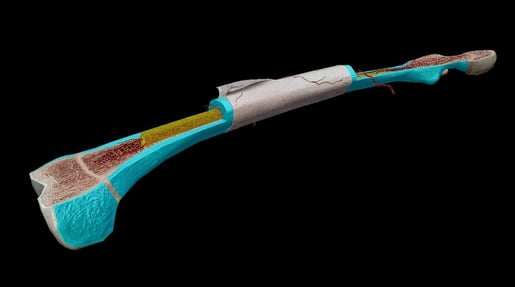This digitally created image depicts a cross-section of a bone-like object, merging elements of anatomical structure and abstract art. The bone is partially cut in half, displaying its internal and external layers in a strikingly detailed manner. The outer surface is predominantly turquoise blue with patches of white, characterized by fine cracks and scratchy brown textures, giving it a weathered appearance. The cut surface reveals a vibrant orange interior interspersed with yellow tubing, simulating marrow or vascular elements. The top of the image showcases the cross-section's flat surface, while the middle tubular part remains intact and fully rounded. The environment around the bone is stark black, providing a sharp contrast that highlights the vivid colors and intricate details of the bone's layered structure. This composite illustration blends anatomical accuracy with artistic interpretation, presenting a fascinating study of a bone's composition and internal complexity.